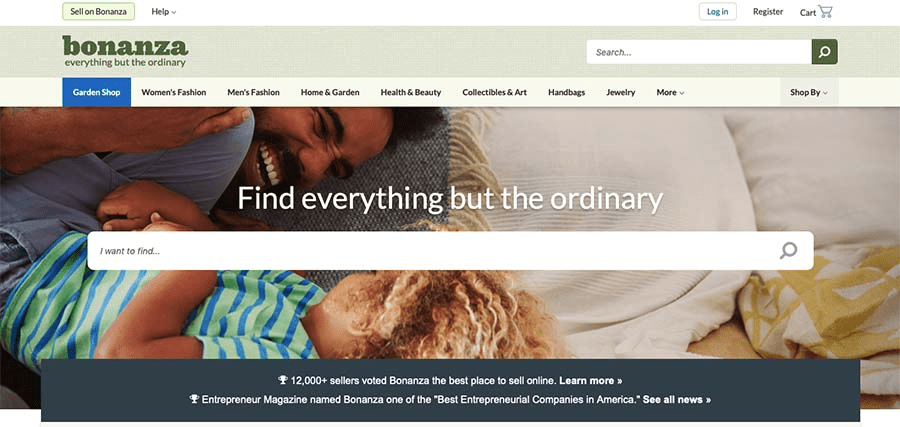The image depicts the Bonanza website, which appears reminiscent of e-commerce platforms like eBay. Prominent colors include green for the logo, darker hues of black for some text, and dark blue elements. The tagline "Bonanza: Everything but the ordinary" is prominently displayed, along with various shopping categories such as "Women's Fashion," "Men's Fashion," "Home and Garden," "Health and Beauty," "Collectibles and Art," "Handbags," and "Jewelry."

The upper right-hand corner features options for "Login," "Register," and an icon for the shopping cart, with "Login" encased in a distinct rectangle, suggesting it is an interactive button. On the left side, the text "Bonanza" is also enclosed in a colorful square, further emphasizing its branding. The website boasts over 12,000 sellers and promotes itself as "the best place to sell online." The user viewing the page is not logged in, as indicated by the presence of the "Login" option.